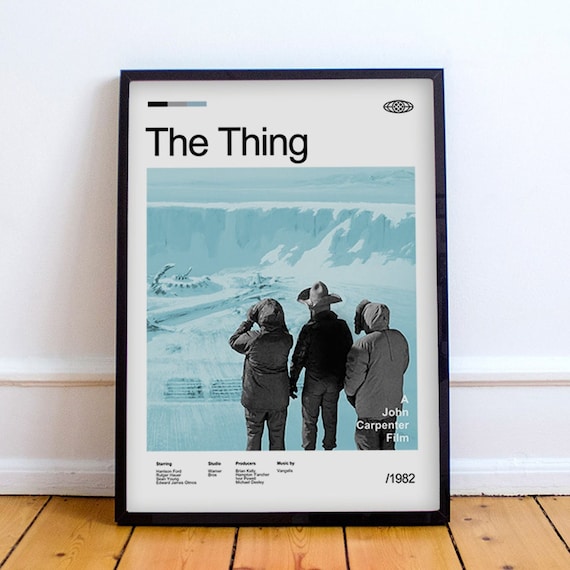The image captures a vertically oriented, framed vintage movie poster for the 1982 film "The Thing" directed by John Carpenter. The poster is enclosed in a black frame with a narrow white mat and leans against a white wall with white trim, set atop a light-colored hardwood floor. Dominated by hues of gray, blue, and black, the central image depicts three men dressed for winter with their backs to the viewer. The man on the left is using binoculars, the center man wears a cowboy hat, and the man on the right has his jacket hood up. They are all gazing towards a snow-covered structure that appears to be inoperable, suggesting an Arctic setting. At the poster’s top left corner, three bars in black, gray, and blue are aligned together, and across the top, the title "THE THING" is displayed in bold black text. The lower right corner has white text that reads "a John Carpenter film," followed by "1982" in black text. Below this, there are additional credits in small, illegible font. The poster's style is photographic with elements of realism, evocative of classic horror-themed vintage film posters.